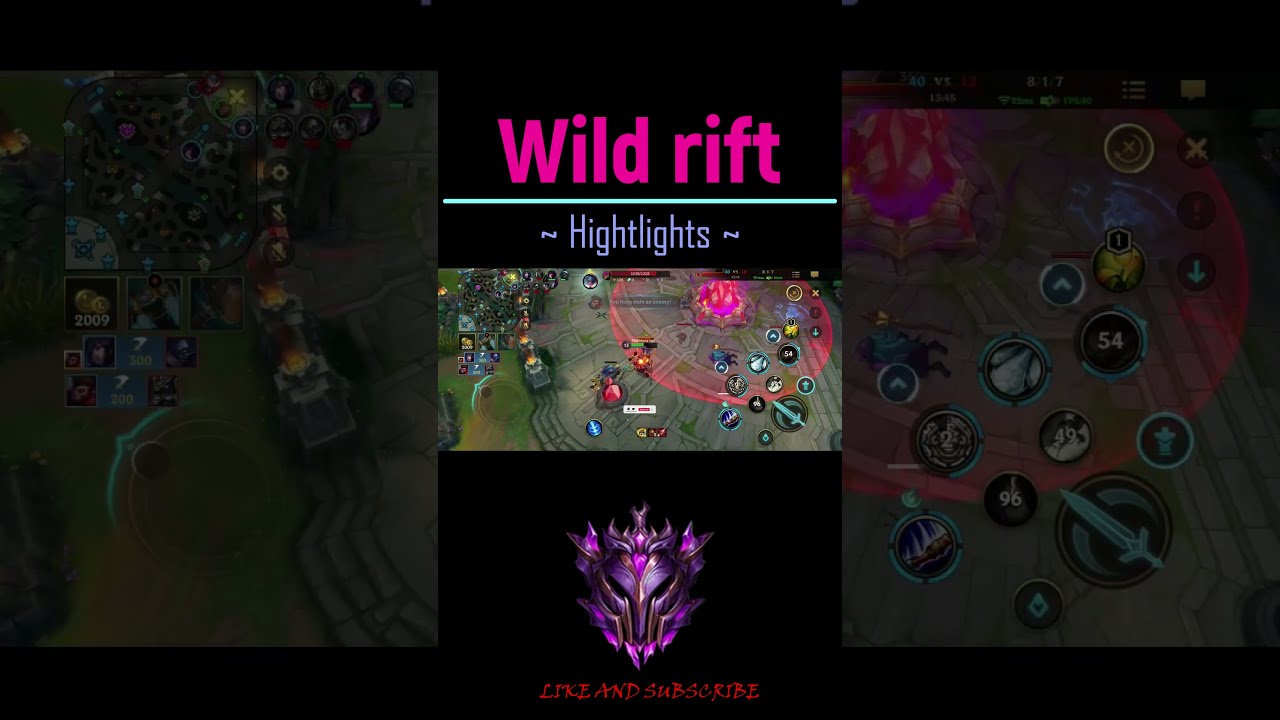The image depicts what appears to be a vibrant and detailed screenshot from a real-time strategy (RTS) mobile game, designed as if for a social media post. At the top, a bold black header spans the width of the image, featuring the words "Wild Rift" in prominent hot pink lettering, followed by a thin light blue line underneath, and "Highlights" written in light blue. The center portion showcases a busy, colorful screenshot of the game, filled with various buttons and characters, seemingly involved in online strategic play. Dominating the middle of the gameplay scene is a red and purple altar, emitting a glowing red light. The sides of the image have been darkened and enlarged excerpts of the game’s screenshot, creating a layered effect. The bottom section includes another black band where a purple and gold-toned mask is displayed. Below this mask, the words "Like and Subscribe" are prominently featured in bright red font.